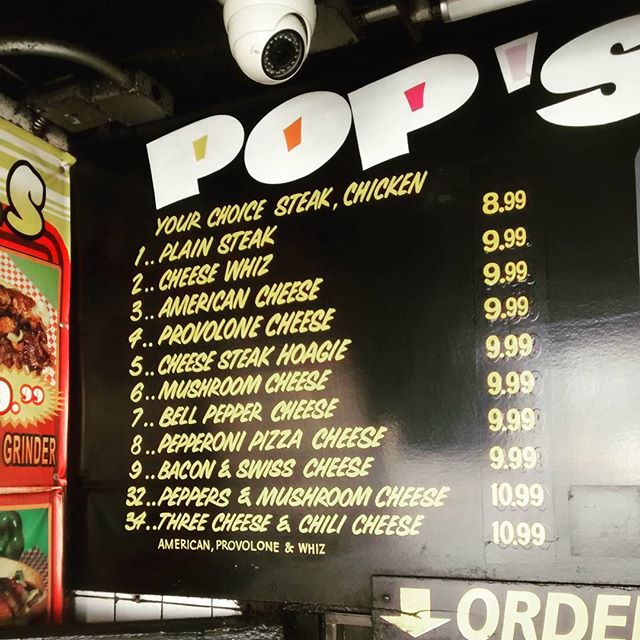This image features a restaurant menu from a place called "Pops." The top text has "Pops" written in white font, while each letter 'P' and the 'O' are creatively designed with yellow, orange, and pink hues, resembling a target or a "hole." Attached to one of the letters is an illustration of a light pink drink.

Below the establishment's name, the main menu items are listed in yellow text as follows:

1. **Plain Steak:** $8.99
2. **Cheese Steak:** $9.99
3. **American Cheese Steak:** $9.99
4. **Provolone Cheese Steak:** $9.99
5. **Cheese Steak Hoagie:** $9.99
6. **Mushroom Cheese Steak:** $9.99
7. **Bell Pepper Cheese Steak:** $9.99
8. **Pepperoni Pizza Cheese Steak:** $9.99
9. **Bacon and Swiss Cheese Steak:** $9.99
10. **Peppers and Mushroom Cheese Steak:** $9.99
11. **Three Cheese and Chili Cheese Steak:** $10.99 (featuring American, Provolone, and another cheese)

To the left side of the menu, there's a visual depicting a "Grinder" sandwich, and an arrow pointing to a phrase that reads "Where quality meets flavor." At the very top of the image, there's a white security camera with a black lens, emphasizing safety and security within the restaurant.